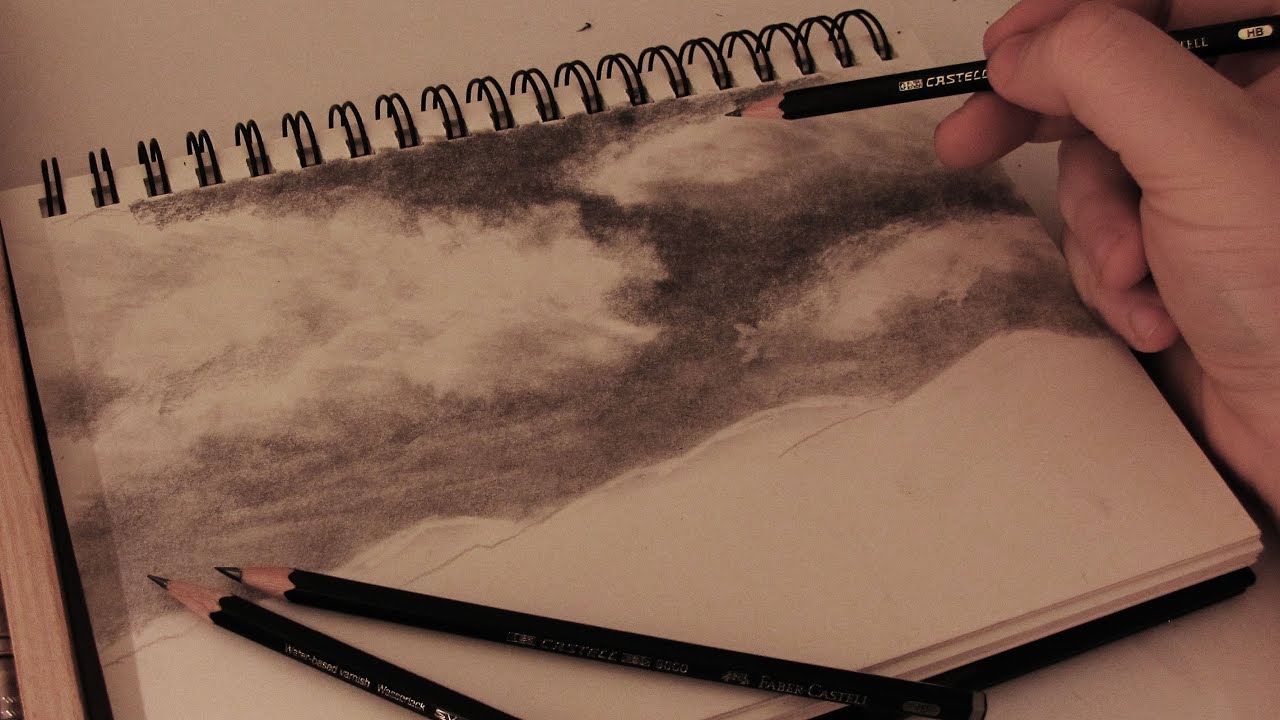This photograph showcases a detailed scene of someone's sketching process. In the top right corner, a right-handed individual, presumably Caucasian, is seen holding a black pencil adorned with gold lettering that partially reads "C-R-S-T-E-C." The sketchbook, which is notably thick and spiral-bound, lays on a white table and is propped slightly to the left against a wooden piece. Alongside the actively used pencil, two other pencils rest on the spiral sketchpad. 

The center of attention is the ongoing sketch, which vividly portrays a landscape. The composition features rolling hills at the bottom, uncolored as the artist seems primarily occupied with the intricate, stormy sky. The sky is filled with dark, wispy clouds that convey a turbulent atmosphere, potentially in black and white, suggesting either an impending storm or one that is dissipating. Despite the incomplete nature of the hills, the sketch gives off a sense of depth and impending weather drama, highlighting the artist’s focus on atmospheric details.